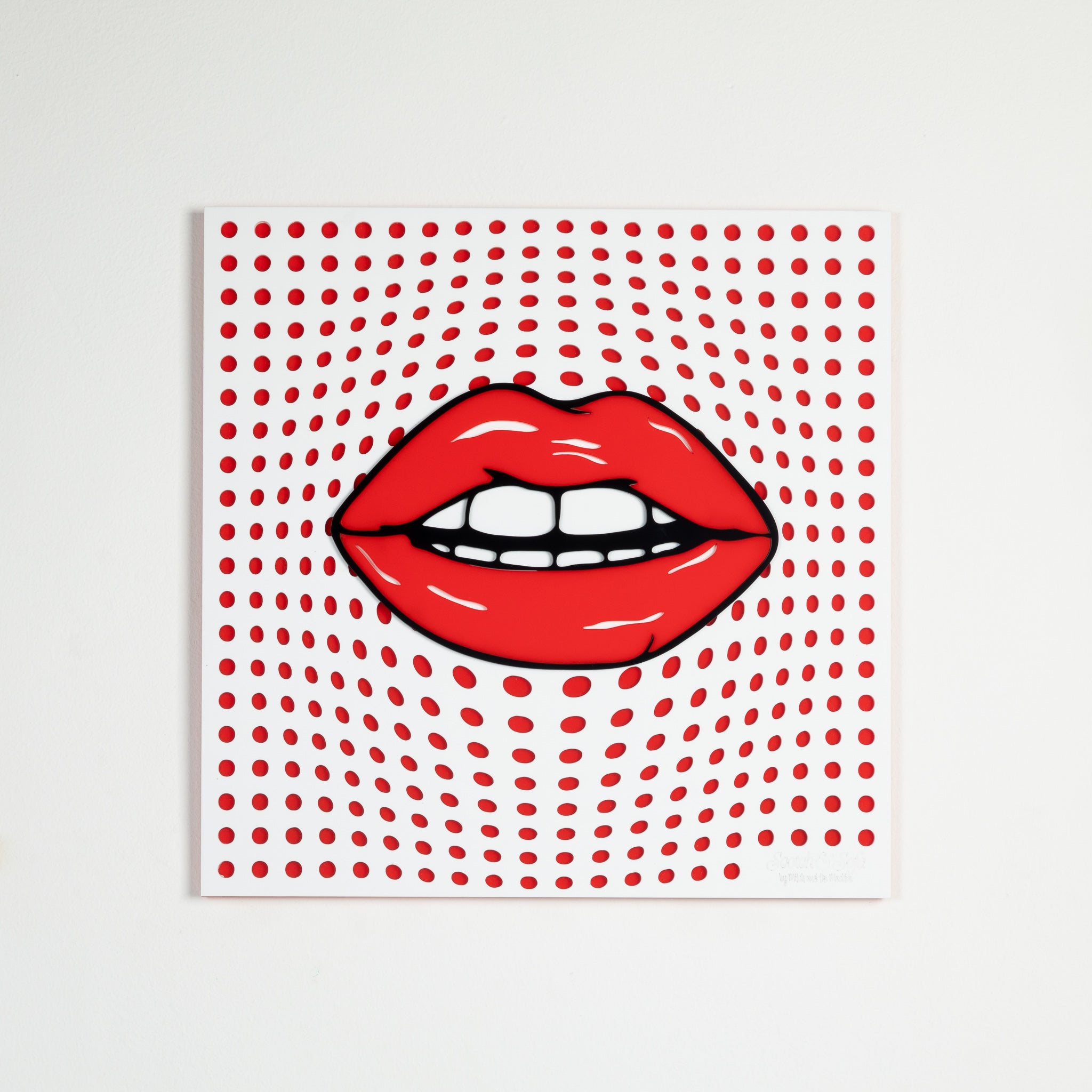This image showcases a captivating piece of artwork set against a light gray wall. The artwork itself is square-shaped and presents a striking graphic depiction of glossy, bright red lips prominently positioned in the center. The lips are slightly parted, revealing both the upper and lower rows of white teeth, which are detailed with thin black lines running through their centers. Enhancing the realism, the lips are rendered with a thick black outline and glossy highlights that add dimension.

The background of the artwork is a meticulously arranged grid of evenly spaced red dots, creating a consistent pattern. This grid, resembling a 20 by 20 array, appears to stretch and distort around the lips, giving a compelling 3D effect: the dots flare outward near the mouth, creating an illusion that the lips are nearly bursting from the surface or engaged in conversation. Overall, this striking interplay of vibrant red elements and dynamic dot pattern evokes a sense of motion and depth, making the lips seem to actively push forward off the canvas.